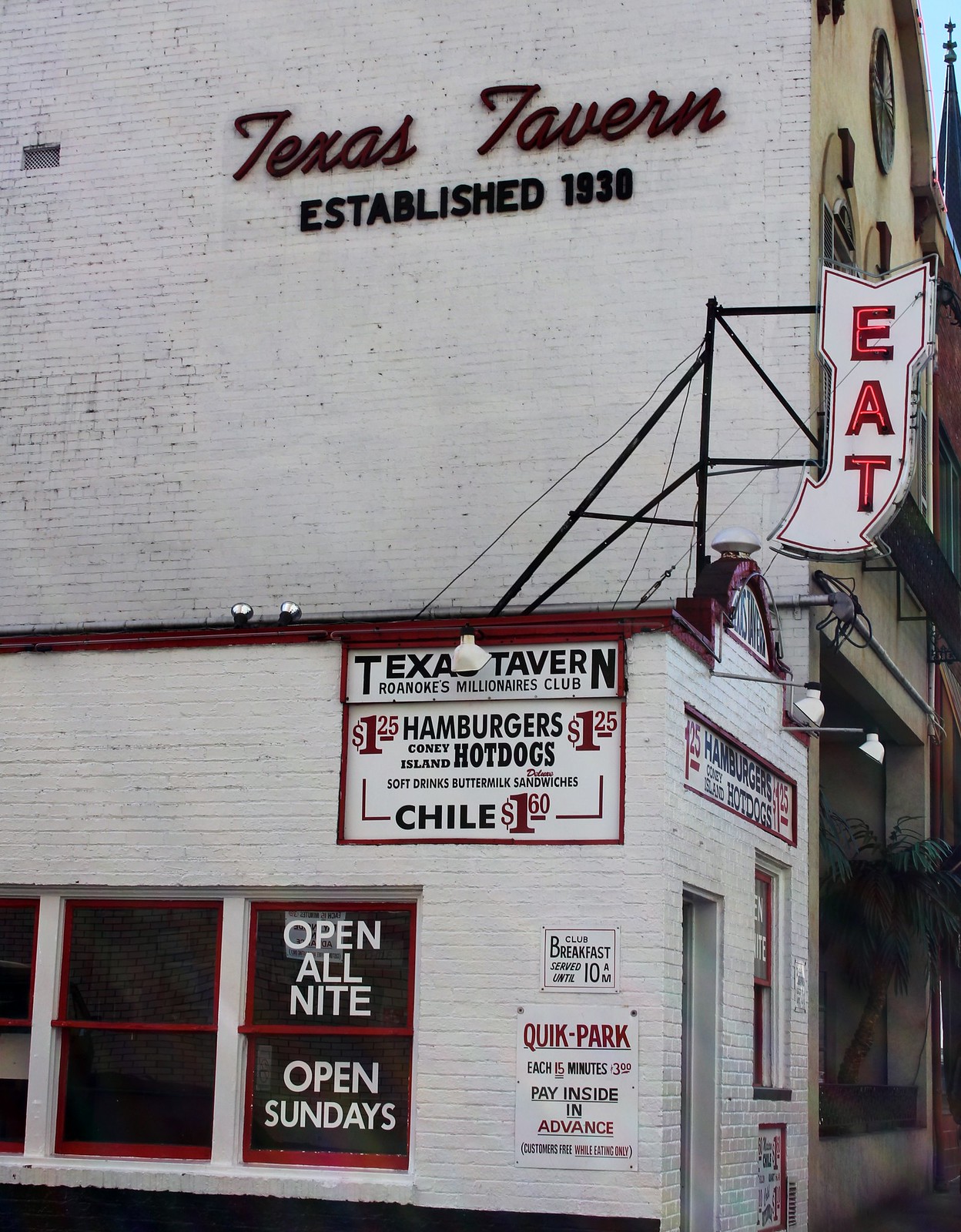The image captures the exterior of a small, single-story white brick restaurant with red trim, named Texas Tavern. The restaurant, with its distinctive cursive signage, "Texas Tavern," and "Established 1930," contrasts sharply with the adjacent multi-story buildings. Dominating the left side of the photo, the restaurant wall is decorated with enticing and nostalgic advertisements: $1.25 hamburgers, Coney Island hot dogs, soft drinks, buttermilk sandwiches, and chili for $1.60. An "EAT" sign with an arrow extends from the roof, inviting passersby. Seen through its windows, more signs proclaim "Open all night, open Sundays." Smaller signs near the front declare, "Club breakfast served until 10 a.m." and parking instructions: "Quick park each 15 minutes, $3. Pay inside in advance. Customers free while eating only." A portion of blue sky and part of a church spire peek from the top right corner, adding to the quaint, urban feel of the setting.